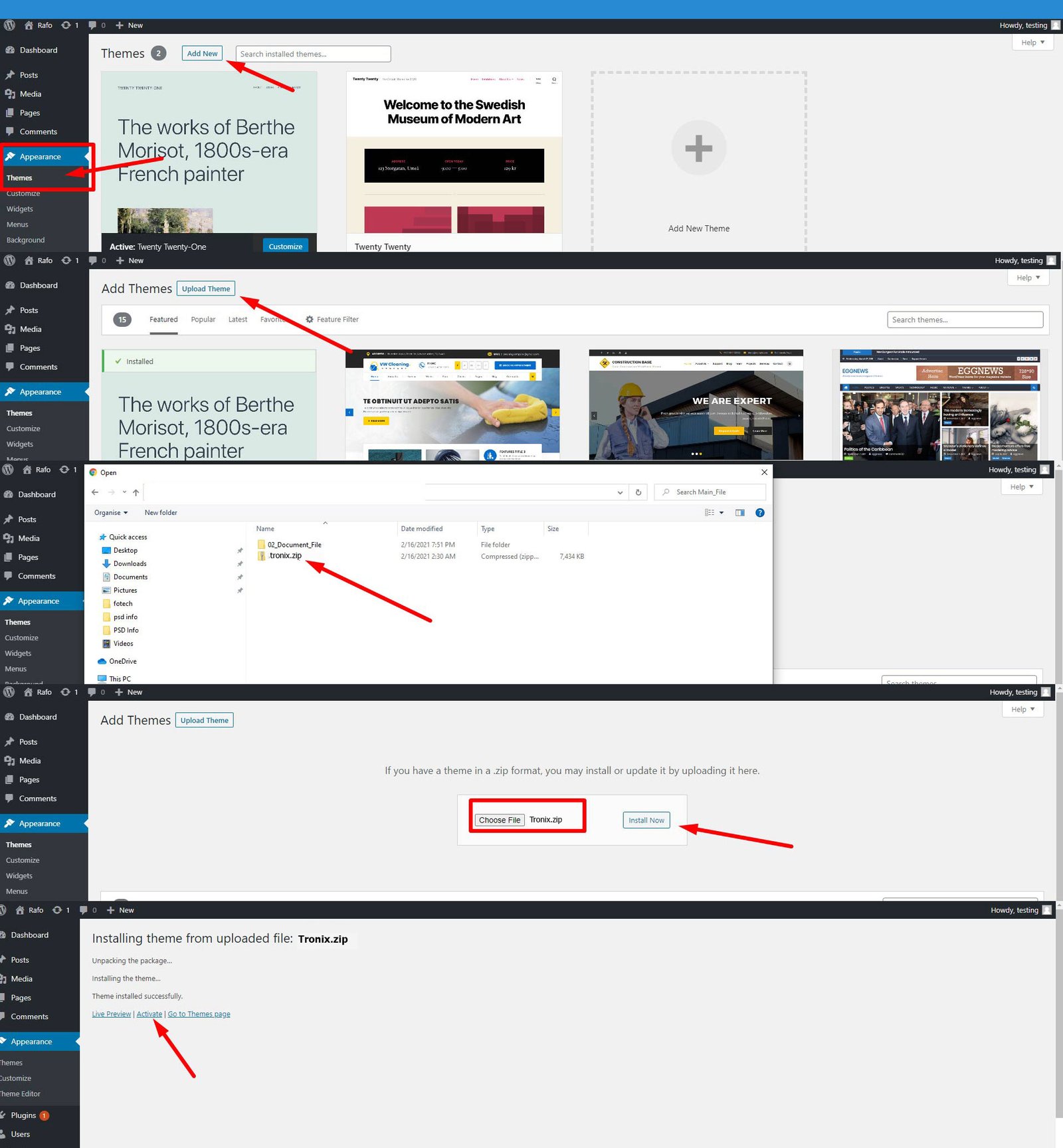In this image, we observe a highly zoomed-out view of a website. The topmost part of the design features a narrow horizontal band with a blue background stretching from side to side. On the left side of the page, multiple categories are displayed vertically. These categories are set against backgrounds that alternate between black and gray squares, and the text within these squares is white. There are numerous options listed, with five of them highlighted in blue. A red rectangle outlines one of these options towards the top of the list.

On the right side of the image, the content is divided into five individual sections, separated by thin black borders. Each section has a light gray background. From top to bottom, the sections are labeled: "Themes," "Add Themes," "Add Themes" (again), and "Installing Themes." Within these sections, various square images are present. The middle section contains an image resembling a file page on a computer. In the bottom section, there are two options, one of which is highlighted by a red rectangle. Each of these five sections also includes a red arrow pointing diagonally to the left.